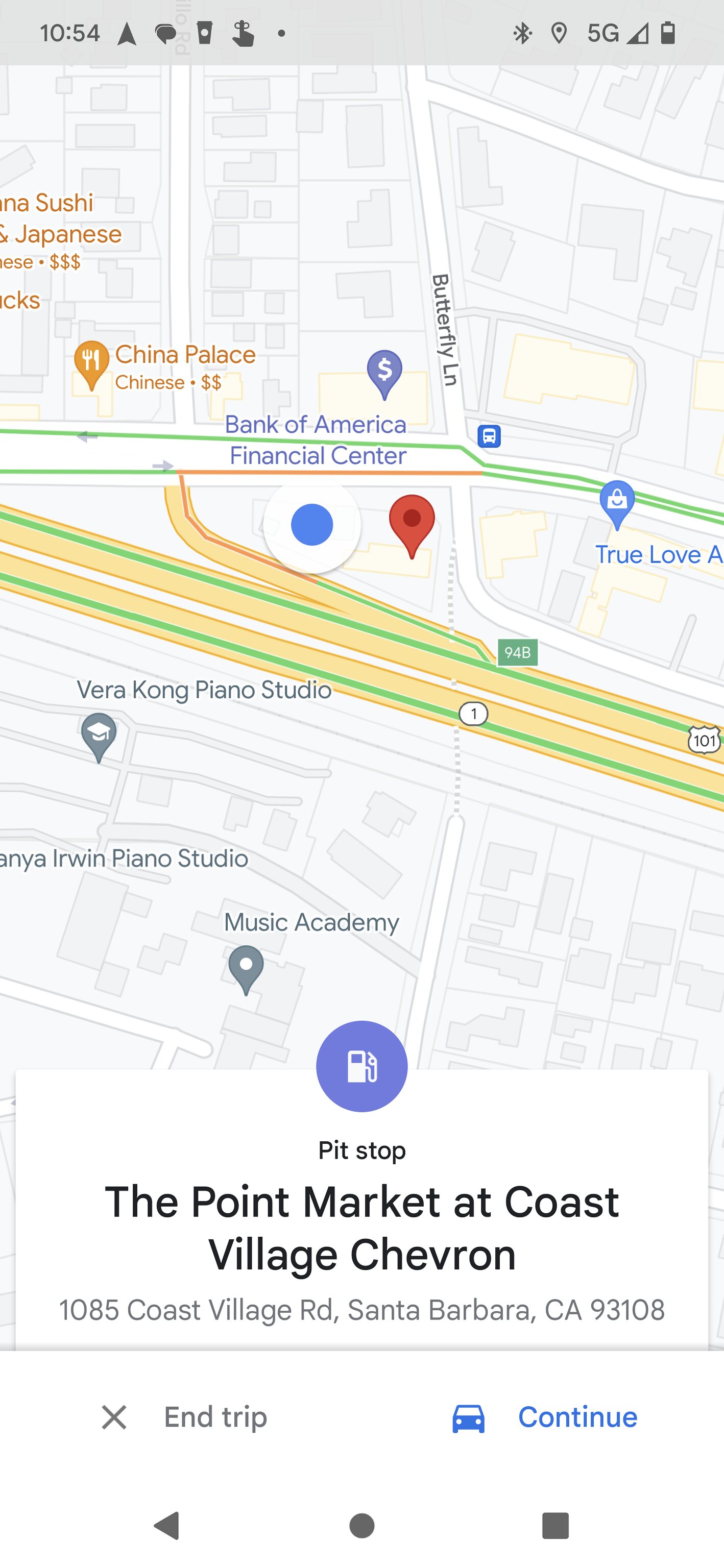This is a detailed photograph of a navigation screenshot, likely taken on an iPhone. The screen displays various points of interest and navigation elements. At the bottom of the screen, the options "End Trip" and "Continue" appear, with "End Trip" on the left and "Continue" in blue on the right. Just above these options, there is a "Pit Stop" label accompanied by an icon depicting a gas pump and a weight, indicating a stop at "The Point Market at Coast Village Chevron," located at 1085 Coast Village Road, Santa Barbara, California 93108.

Higher up on the screen, a teardrop pin marker is labeled "Music Academy." Further up, two more locations are marked: "Irwin Piano Studio" and "Vera Kong Piano Studio." A prominent highway, labeled 101, is displayed in tan with green edges.

A red teardrop pin indicates the location of "The Point Market." To the left of this pin, a white circle with a blue dot marks the user's current location. Above this marker, "Bank of America Financial Center" is noted, close to another teardrop pin with a dollar sign, likely representing another Bank of America location.

Further details include a teardrop pin with a fork and knife icon labeled "China Palace, Chinese," and the word "money." Additionally, there is another pin labeled with "sushi" and "Japanese," also accompanied by money signs. At the top left of the screen, a label reads "1054," surrounded by a series of smaller icons and graphics, indicating various businesses and services in the area.